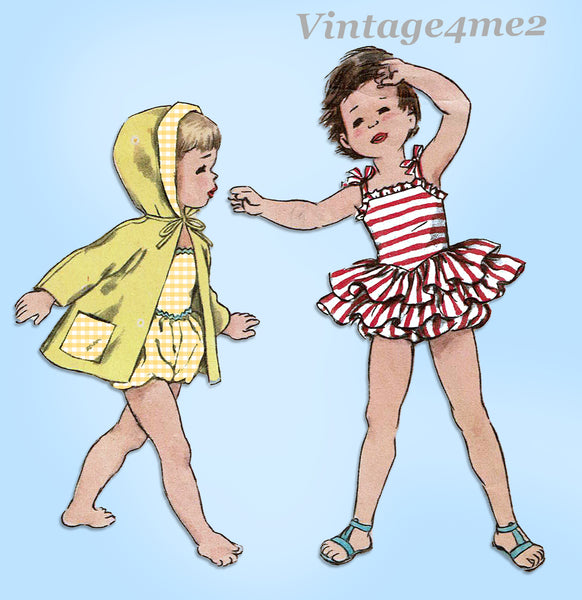This image is a square, approximately four inches by four inches, with a light blue background. In the upper right-hand corner, bold brownish-tan text reads "vintage 4ME2," with the numbers 4 and 2 in numeral form. Below the text, there are illustrated drawings of two young girls showcasing vintage children's outfits, resembling a 1950s advertisement.

The girl on the left appears to be around three to five years old, with Caucasian skin and blonde hair, and is depicted walking from left to right. She is dressed in a retro yellow and white checkered romper with a coordinating yellow raincoat. Her raincoat has pockets and a hood lined with the same yellow and white checkered pattern as her romper.

The girl on the right appears slightly older and taller, and has short black hair styled in a way that gives the impression it’s being tousled by the wind. She is shown in a white and red striped sundress with blue sandals. Her dress has a vintage charm, resembling a ballerina-style outfit or a bathing suit with ruffles at the bottom, possibly hinting at an American flag theme with its red, white, and blue colors. One of her arms is lifted near her head, while the other is outstretched to the side.